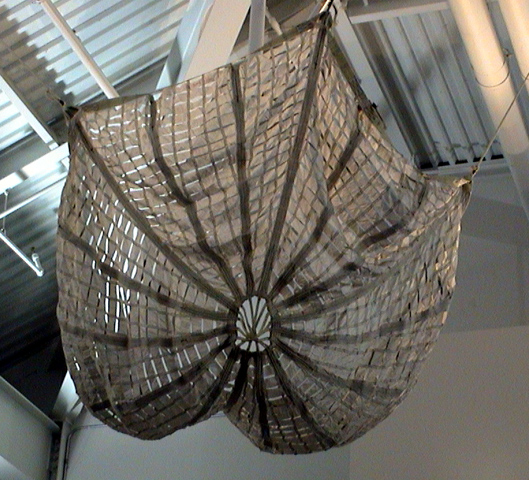This photograph depicts an intricate, suspended fabric installation, evocative of an inverted parachute or umbrella, within a warehouse-like setting with a metallic, light blue and white ceiling. The structure is composed of light gray cloth with straps extending from a central open circle, creating a spider web effect with additional straps forming a grid between these branches. Secured by approximately six hooks, the fabric is attached to the ceiling beams and pipes by ropes. The arrangement is punctuated by slits between the fabric sections, which allow light to pass through, creating an ethereal effect. The setup gives an impression of a large, delicate sea urchin or a hammock-like entity, enhanced by the industrial surroundings of beams and rods.